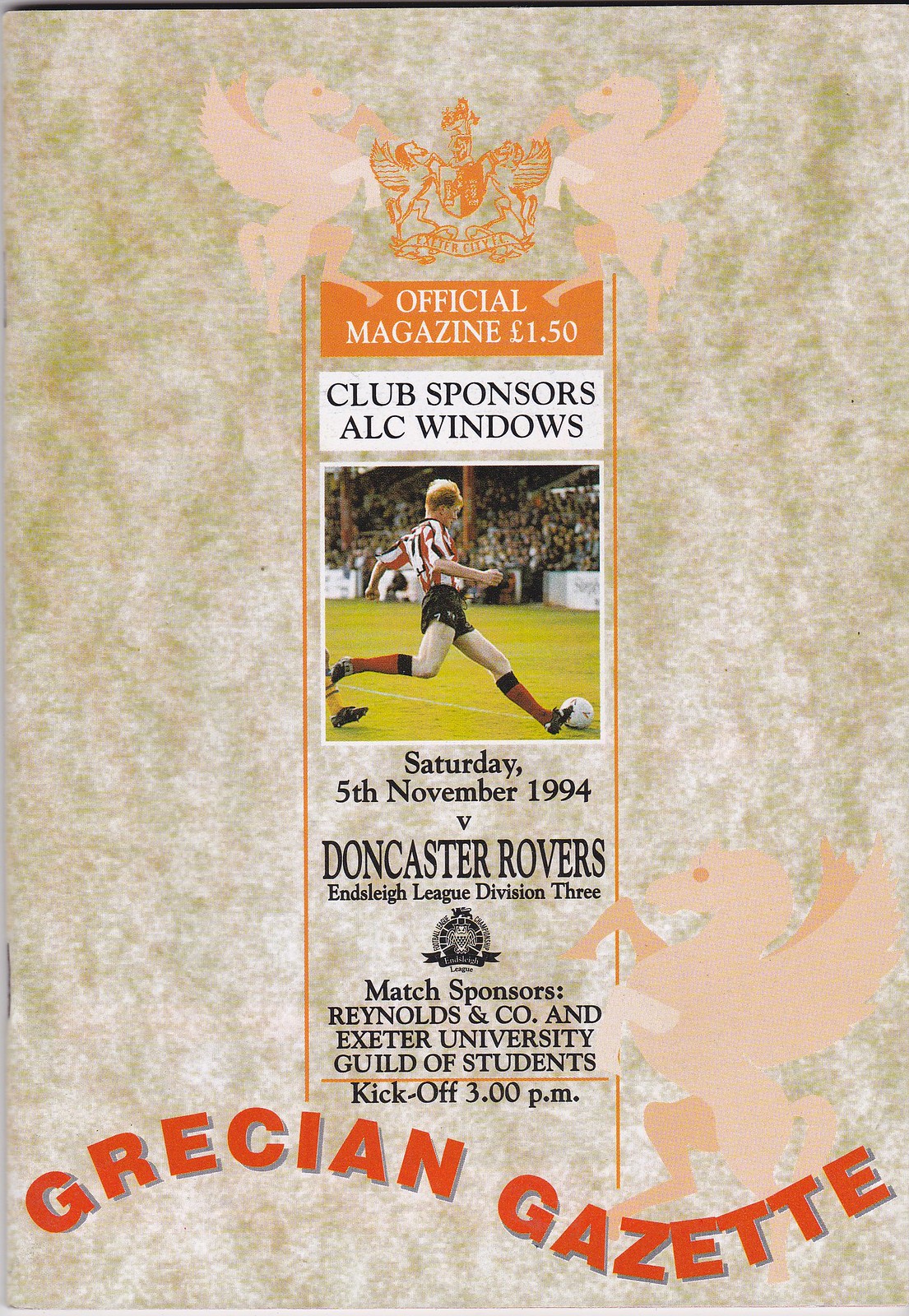This is a detailed cover image of a football program from the "Grecian Gazette." The background features a mottled, off-white, greenish, rose pattern, giving it a hazy, almost carpet-like appearance. There are two orangey-cream colored Pegasus figures, one on each side of an orange crest that is adorned with unicorns. In the top center, small white text on the orange crest reads "Official Magazine, £1.50." Below this, the text "Club Sponsors, ALC Windows" is displayed in black within a white box. 

Central to the cover is a rounded rectangular photograph of a football player running down the field, dressed in a white and red jersey. Beneath the image, in black text, it reads "Saturday, 5th November 1994, versus Doncaster Rovers, Endsleigh League Division III, Match Sponsors: Reynolds and Company, and Exeter University Guild of Students, kickoff 3 p.m." The program title, "Grecian Gazette," is written in an orange, wavy pattern at the bottom. The overall design conveys a sense of tradition and excitement surrounding the featured football match.